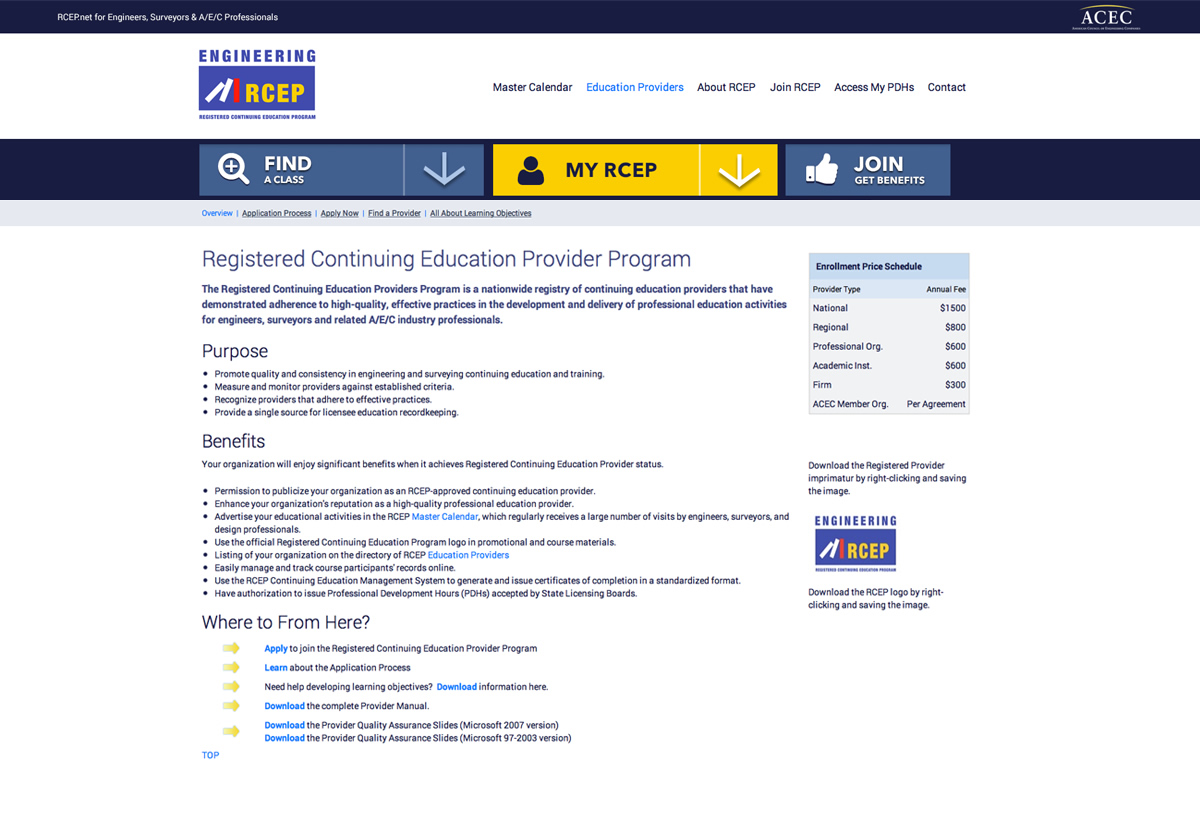### Caption for the Image:

This image features the website design of the Registered Continuing Education Provider (RCEP) Program, a resource for engineers, surveyors, and AEC (Architecture, Engineering, and Construction) professionals. 

1. **Header and Logo**: In the upper right-hand corner, the logo of ACEC (American Council of Engineering Companies) is displayed with a yellow arc over it, and there's small, unreadable text below.

2. **Main Section**: 
   - **Title**: The word "Engineering" is prominently displayed in large blue letters.
   - **Visual Element**: A blue box with a bluish-purple hue containing three books—two white and one red—leaning into each other.
   - **Text**: Beneath this, "RCEP" appears in yellow text.

3. **Navigation Menu**: 
   - **Options**: Master Calendar, Education Providers (highlighted in blue as the current selection), About RCEP, Join RCEP, Access My PDHs, and Contact.
   - **Additional Buttons**: A button labeled "Find a Class" and a yellow box with "My RCEP" and an icon of a person next to a down arrow in white.
   - The "Join, Get Benefits" button features a thumbs-up icon.

4. **Content Description**:
   - **Program Overview**: The "Registered Continuing Education Provider Program" (RCEP) description, emphasizing quality, consistency, and the recognition of effective practice in professional education for engineers, surveyors, and AEC professionals.
   - **Program Purpose**: Four bullet points explain the goals, including promoting quality, consistency, monitoring providers, and providing a centralized record-keeping source.
   - **Benefits Section**: Outlined with bullet points, detailing how organizations can publicize their RCEP status, enhance their reputation, advertise on the master calendar, and manage educational records online.

5. **Application Process**:
   - A section titled "Where to from here," with five yellow arrows guiding users to different resources:
     - Apply to join the program.
     - Learn about the application process.
     - Download information on developing learning objectives.
     - Access the complete provider manual.
     - Download quality assurance slides for different Microsoft versions.

6. **Right Sidebar**:
   - **Enrollment Price Schedule**: A chart listing provider types and corresponding annual fees:
     - National: $1,500
     - Regional: $800
     - Professional Organizations: $600
     - Academic Institutions: $600
     - Firms: $300
     - ACEC Member Organizations: Per agreement
   - **Download Instructions**: Guidance on downloading the registered provider logo and the RCEP logo by right-clicking and saving the images.

At the bottom, there is a "TOP" button allowing users to quickly return to the top of the page.